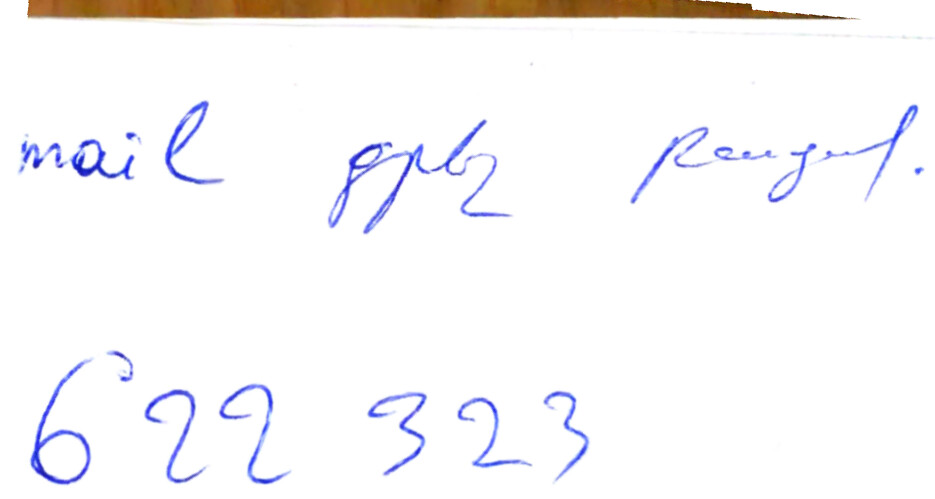The image features a piece of white paper resting on a wooden table. The paper contains text written in blue, italicized letters. The text reads "Male" followed by a drawing labeled "PM2." Below this, the word "Regan" is written, and beneath it, the number "622323" appears. This paper seems to be a quick note, possibly containing contact information or a reference to a person's address.